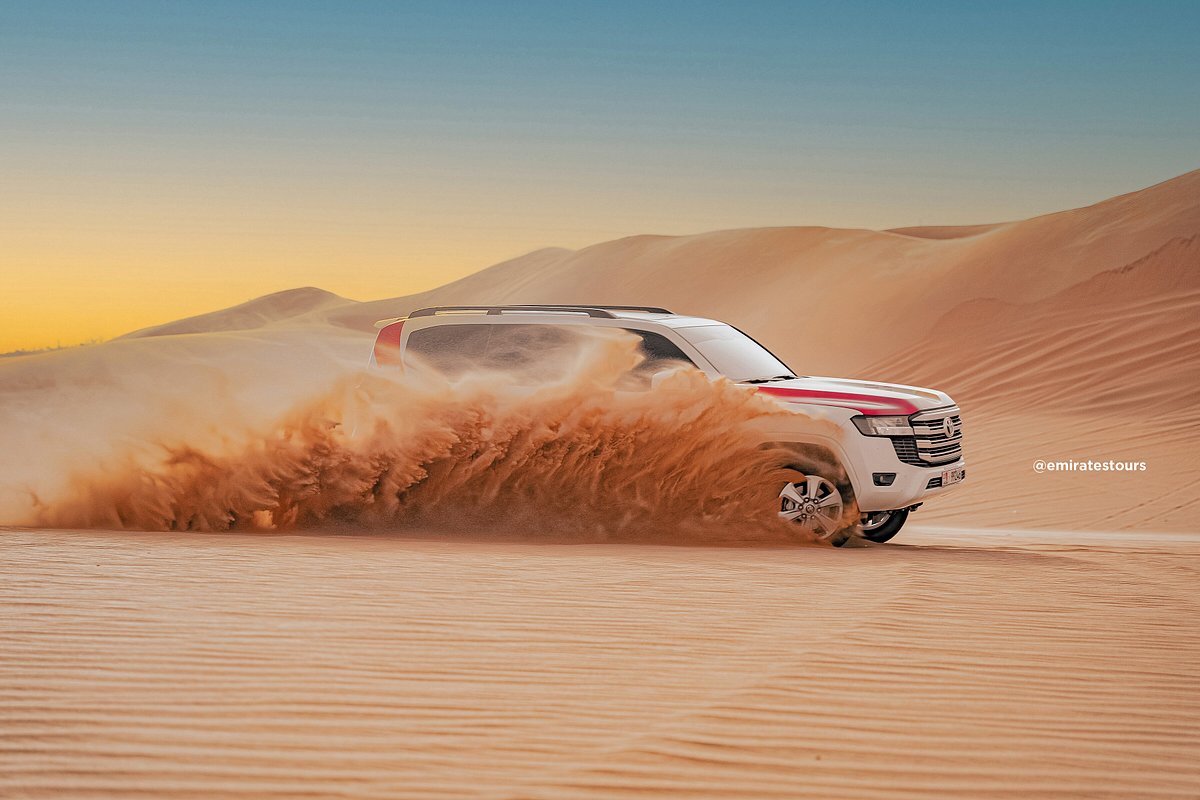In a dynamic and picturesque desert setting, this photograph captures a pristine white SUV with distinctive red stripes racing through wavy sand dunes at either sunrise or sunset. The golden hue of the sun, peeking over the horizon against a clear blue sky, illuminates the scene with a serene glow. The SUV, seen from the right side and partially obscured by a substantial eruption of sand, looks immaculate and undamaged, exuding the polished appeal typical of a car commercial. The foreground shows rippled sand while the background features sloping sand dunes, adding depth and a sense of rugged adventure to the composition. Notably, a white watermark reads "@emirate_tours," suggesting this image might be part of a promotional campaign for desert tours.